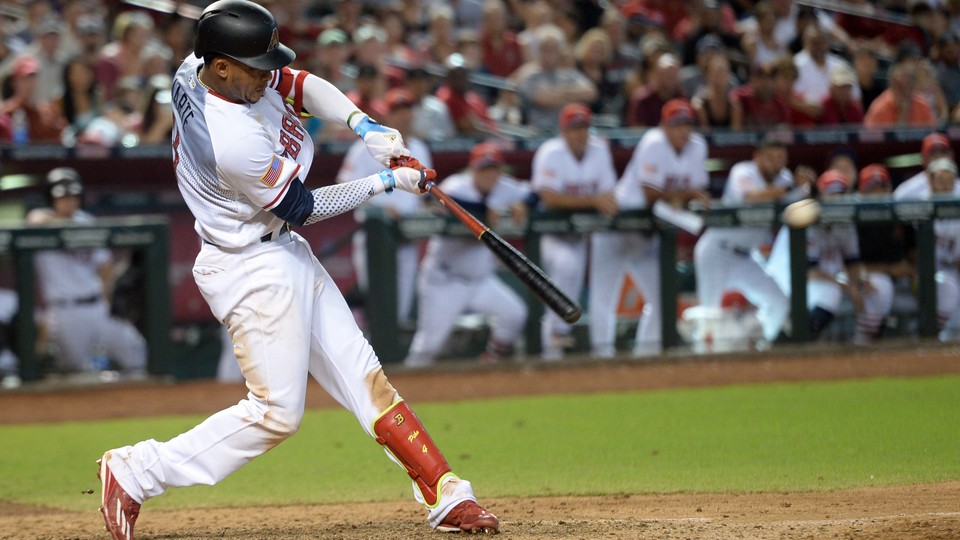A close-up view captures a professional baseball player of African descent in mid-swing on the batting mound, outdoors during the daytime. The player, dressed in a white uniform with red accents and dirt stains on his back and knee, wears red and white shoes and black gloves. His black ball cap, adorned with a letter 'A' and an American flag patch on the sleeve, remains turned forward as he positions his body in a twisted motion. The bat he wields is black with a red-striped handle, pointed towards the ground. The back of his jersey partially reveals the name "ARTE" in black print, while the front displays the letters 'B' and 'A' in red. His extended left leg and bent right leg, set against the brown dirt of the field, lead into the green grass further behind him. In the background, the dugout features teammates in white uniforms and red caps, leaning over the fence in anticipation, as blurred fans fill the stadium seating, capturing the intense moment of the game.